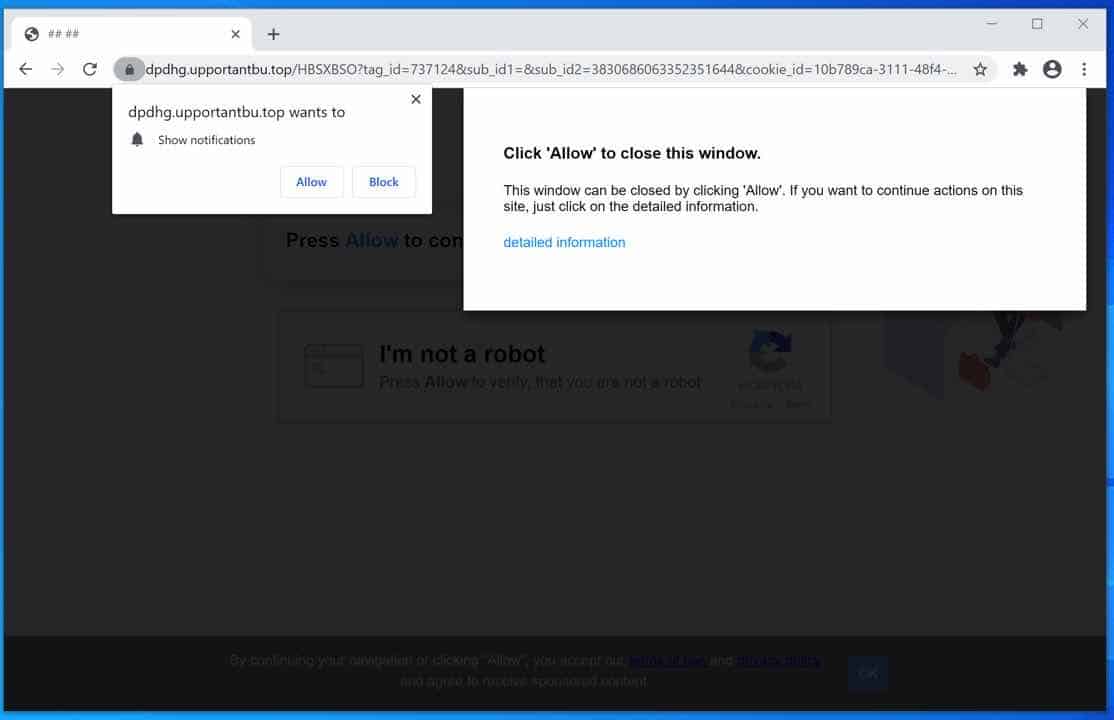The image shows an open web browser, specifically Google Chrome, displayed on the left portion of the screen. The browser window features a single tab with a white background. On the far left of this tab, there is a gray globe icon followed by the placeholder text "####," with spaces in between each pound sign. 

At the bottom of the browser window, a navigation bar is visible. It includes a leftward-pointing gray arrow indicating the 'Back' option, and next to it, a disabled 'Forward' button, signified by its light gray color. To their right, there is a 'Refresh' button represented by a curved arrow. Further to the right, the URL bar contains a lengthy web address.

In the foreground, a notification pop-up is displayed. This rectangular white overlay reads "dpdhg.upportantbu.top wants to," followed by a notification symbol depicted as a gray bell icon. To its right, small gray text reads "show notifications." Below this text on the bottom right, there are two rectangular buttons with shadowy gray borders: a blue "Allow" button and a "Block" button.

Another larger rectangular pop-up appears to the right. It has black bold text stating, "click allow to close this window." Below it, in smaller black text, it reads, "This window can be closed by clicking allow. If you want to continue actions on this site, just click on the detailed information." At the bottom left of this pop-up, a clickable blue text saying "detailed information" is provided.